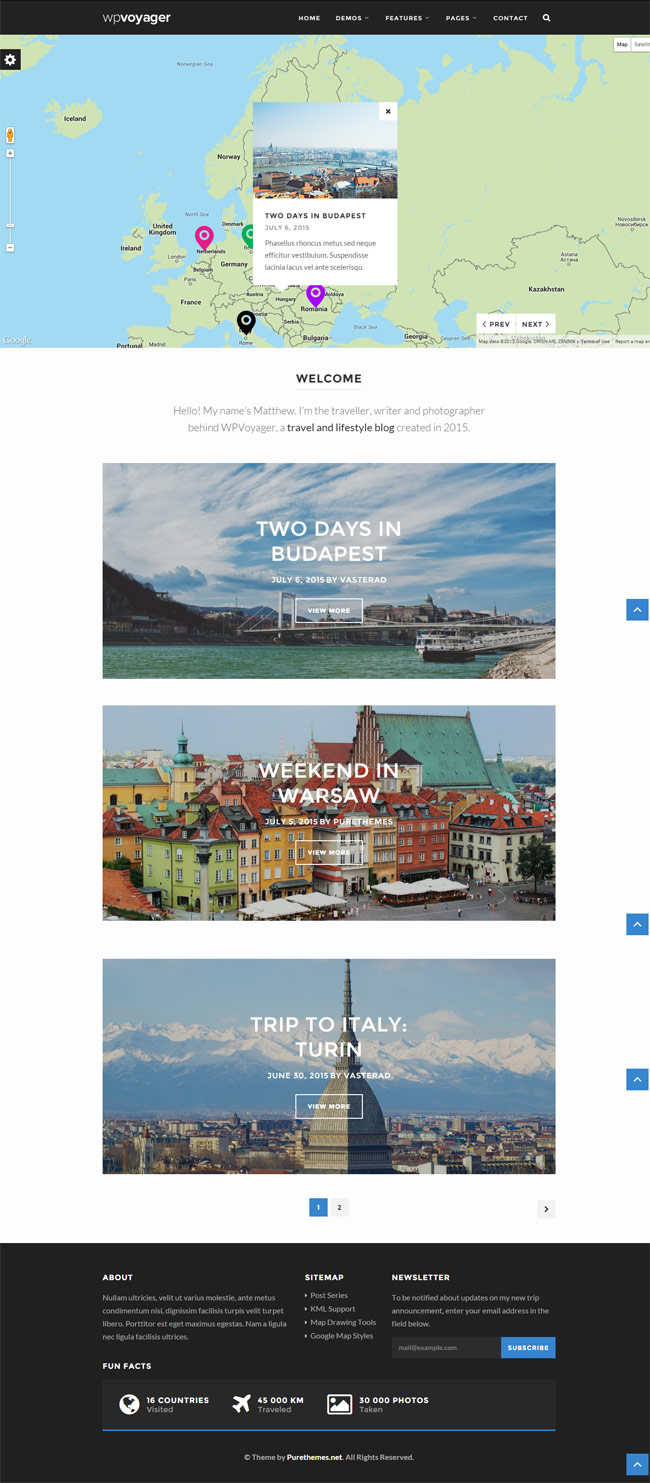A vertical screenshot, possibly from a mobile device, features an organized layout with five distinct rectangles. At the top is a large rectangle displaying a map predominantly showing Europe and Asia. The upper left corner of this rectangle reads "WP Voyager." Superimposed above the map of Europe is a smaller box that states "Two Days in Budapest," followed by detailed text providing further information about this trip.

Underneath this large map section is a smaller rectangle, showcasing an image of water, a boat, land, and the sky. Below this image are three smaller rectangular sections:

1. The first middle rectangle is captioned "Weekend in Warsaw" and portrays a vibrant, colorful town scene.
2. The middle of the three displays "Two Days in Budapest" and contains an image of a charming scene with water and a boat.
3. The last of the three features a striking image of white-capped mountains, clear skies, and a prominent pointy building at its center, captioned "Trip to Italy: Turin."

At the very bottom is a large black rectangle with white text. This section contains general site information, such as an "About" page, site map, and newsletter details, with a prominent blue "Subscribe" button for readers interested in following the travel blog. The text introduces "WP Voyager," a travel and lifestyle blog created in 2015 by Matthew, the traveler, writer, and photographer behind the content.